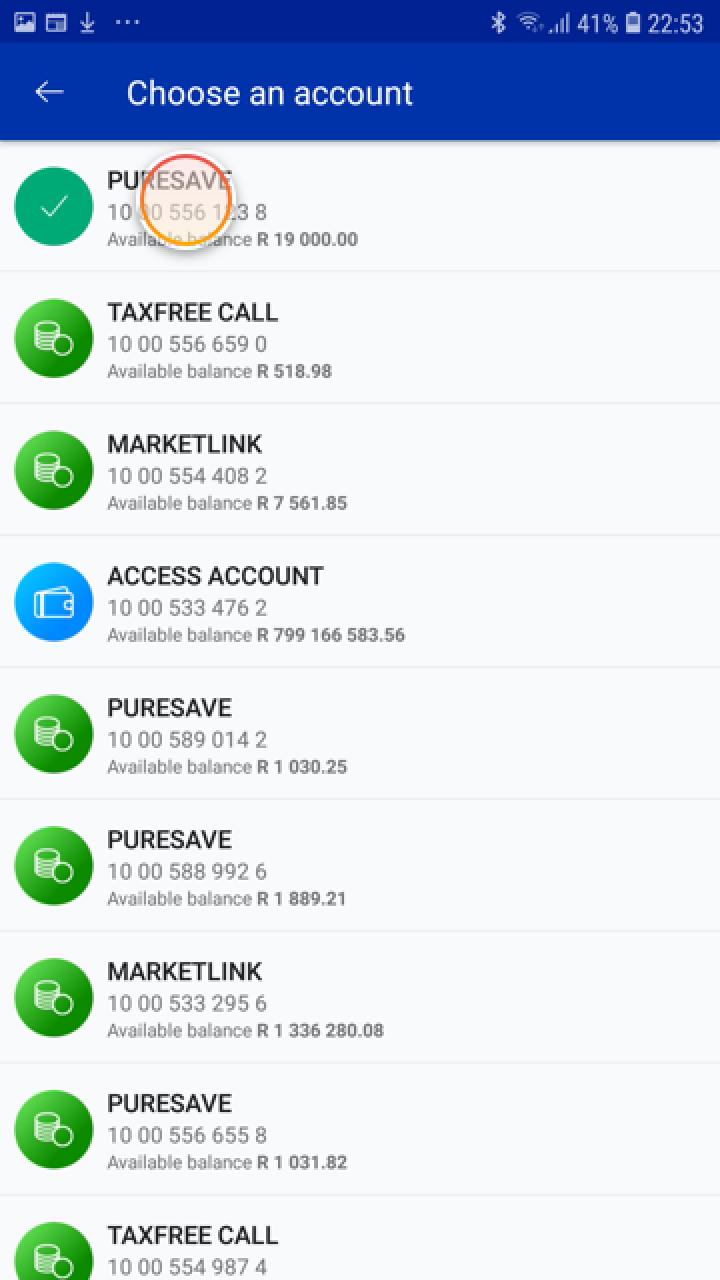In the screenshot depicted, the dark blue header features white icons for a photo gallery, Bluetooth, Wi-Fi, signal strength, and a battery indicator showing 41% charge. The current time is displayed as 22:53. Beneath this header, white text prominently reads "Choose an account" against a gray background.

Displayed below this are several account options: the first being "PureSave" with a green circle containing a white checkmark to the left. Next are "Tax-Free Call" and "Market Link," each in bold black text, also accompanied by green circles on the left.

Further down, there is a blue circle followed by the text "Access account." The available balance for this account shows an extremely detailed figure: 799,166.58356. On the right, within a green circle, the text reads "PureSave," showing an available balance of R1,030.25. Another "PureSave" account is listed below with an available balance of R1,889.21.